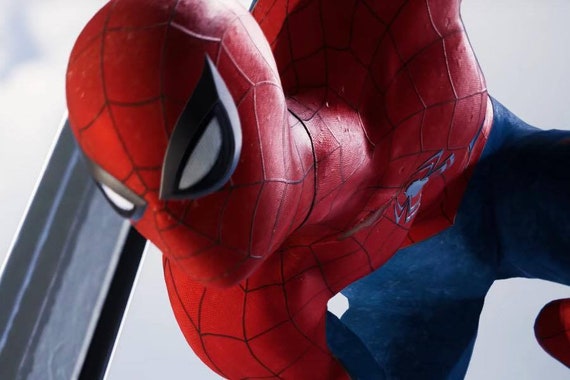This is a close-up image of Spider-Man, capturing the iconic superhero in detailed clarity. The character is prominently displayed with his red face mask featuring black web-like outlines around his large, expressive white eyes, which appear to be squinting slightly as if he's focusing intently. His mask completely covers his face, obscuring his nose and mouth, reflecting the signature design from the Spider-Man comics and movies. The texture of his suit is notable, particularly where the light catches the right side of his neck, revealing a bumpy, ridged surface that suggests a finely crafted figurine or sculpture rather than a live-action shot.

In the image, Spider-Man's head is the main focus, but parts of his neck, chest, and shoulder are also visible, adorned in the familiar red and blue colors of his costume. His blue suit continues from his chest and is partially visible to the right before the frame cuts off. The character seems to be in a posture that suggests he is either hanging or crouched, as if perched on a building, looking downward to his left as though surveying the city below. The background of the image is stark white, with a gray metal board descending on the left side, adding contrast and directing attention to Spider-Man himself.